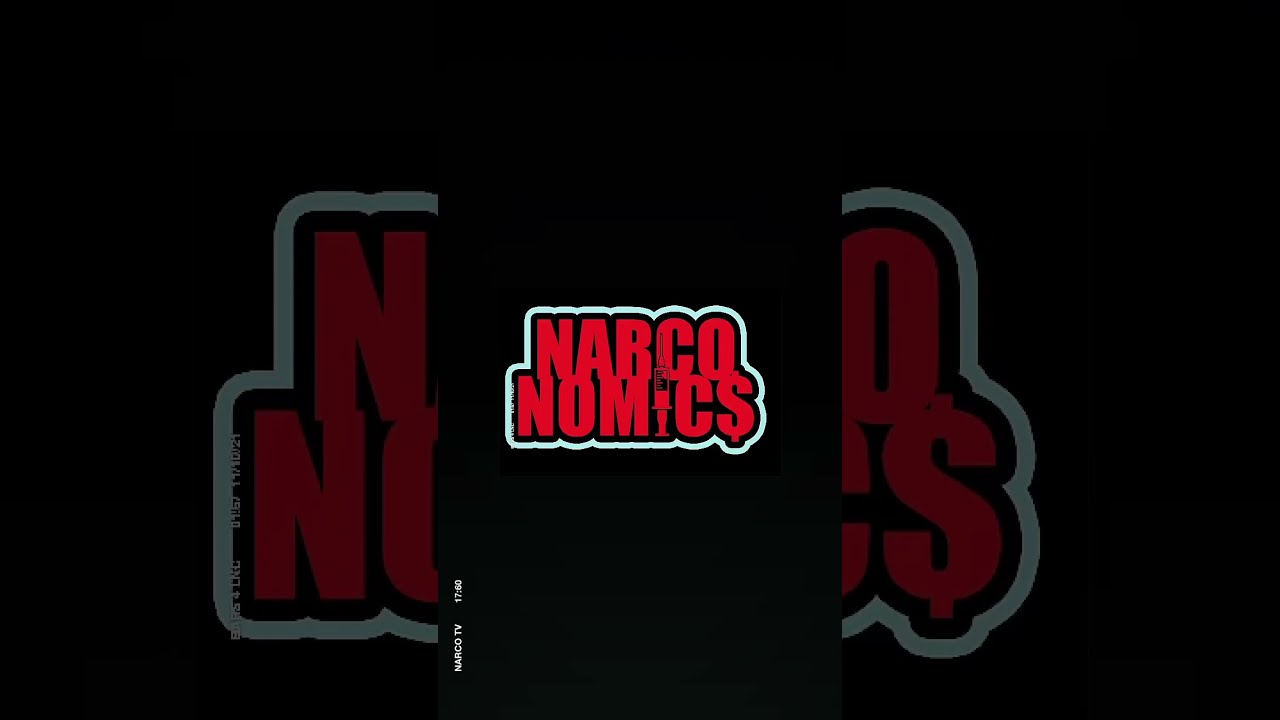The image features a digitally created logo for "Narconomics," centered against an all-black background. The primary text reads "NARCONOMICS" in large, bubble-like red letters with a white outline. Notably, the "I" in "NOMICS" is depicted as a hypodermic needle partially filled with red liquid, emphasizing a possible theme related to drug economics. The "S" at the end of "NARCONOMICS" is stylized as a dollar sign, reinforcing the financial aspect of the theme. Below the primary text, additional smaller text spells out "N-O-M-I-C" in white.

The background of the image is a larger, shaded, and slightly blurred version of the same logo, with overlapping elements such as the red "N" on the left and the intersecting "O" and dollar sign on the right. There is some unreadable white text in the lower left corner. The entire composition is artistic and appears to be part of a digital work or presentation slide, possibly extracted from a webpage or video. The design suggests themes of drug trade and economics, hinted at through the specific visual elements used.